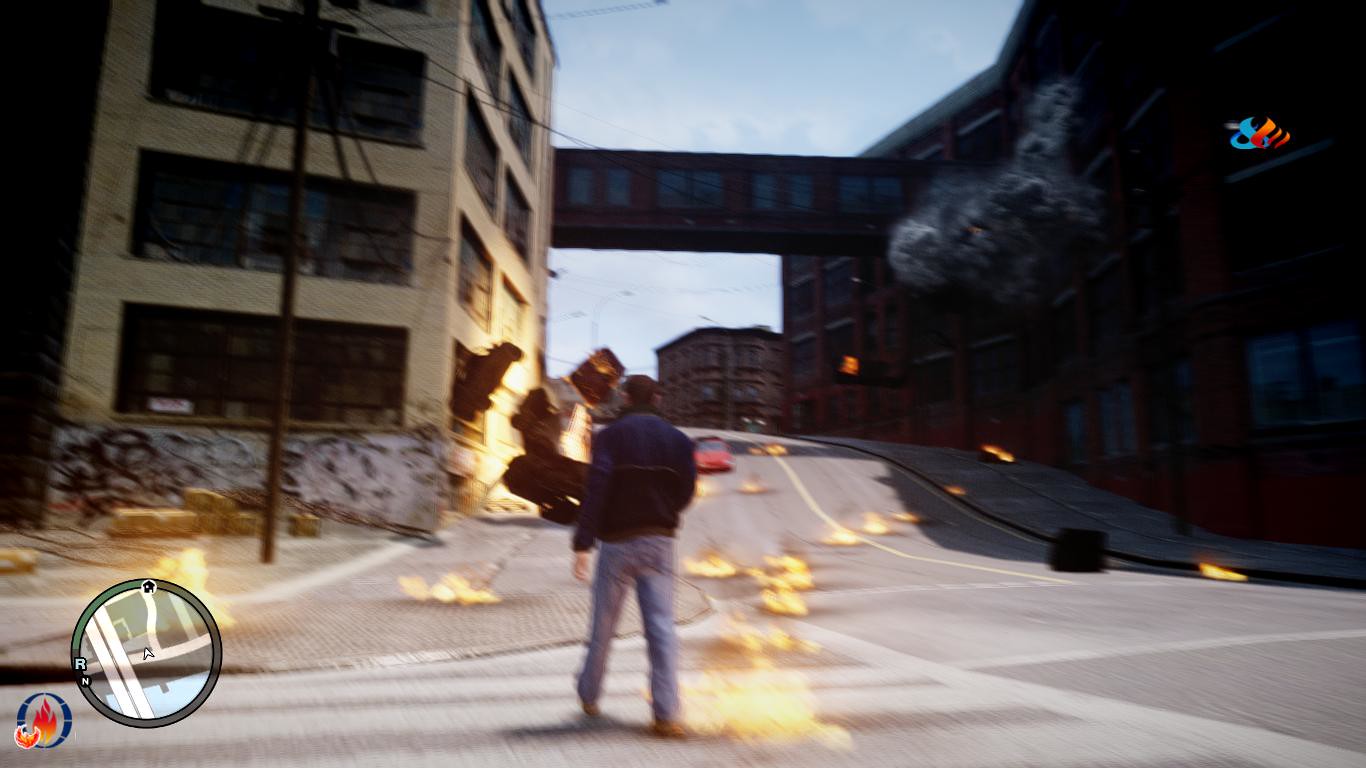In this vivid screenshot from a Grand Theft Auto-style video game, the central figure is a man depicted from the back, walking along a zebra crossing towards the other side of the street. He is clad in a navy-blue jacket over denim jeans, with his right leg and foot stepping forward. The scene is chaotic, with multiple fire spots scattered across the grey street. To the man's left is a building that resembles a storage facility, with cars crashing onto the road from its entrance. Further ahead, a red car is approaching from the opposite side of the street. The cityscape in the background features various buildings, though the details on the right side are obscured by shadows. Contrasting this, the left upper corner showcases a white building with large black rectangles and a beige hue lower down. The sky above is a clear blue with faint white clouds. On the lower left corner of the screen, there is a green circular map indicator displaying the character's position within the city. Additional game elements include a circle inset with red and yellow flames, hinting at in-game activity or objectives.